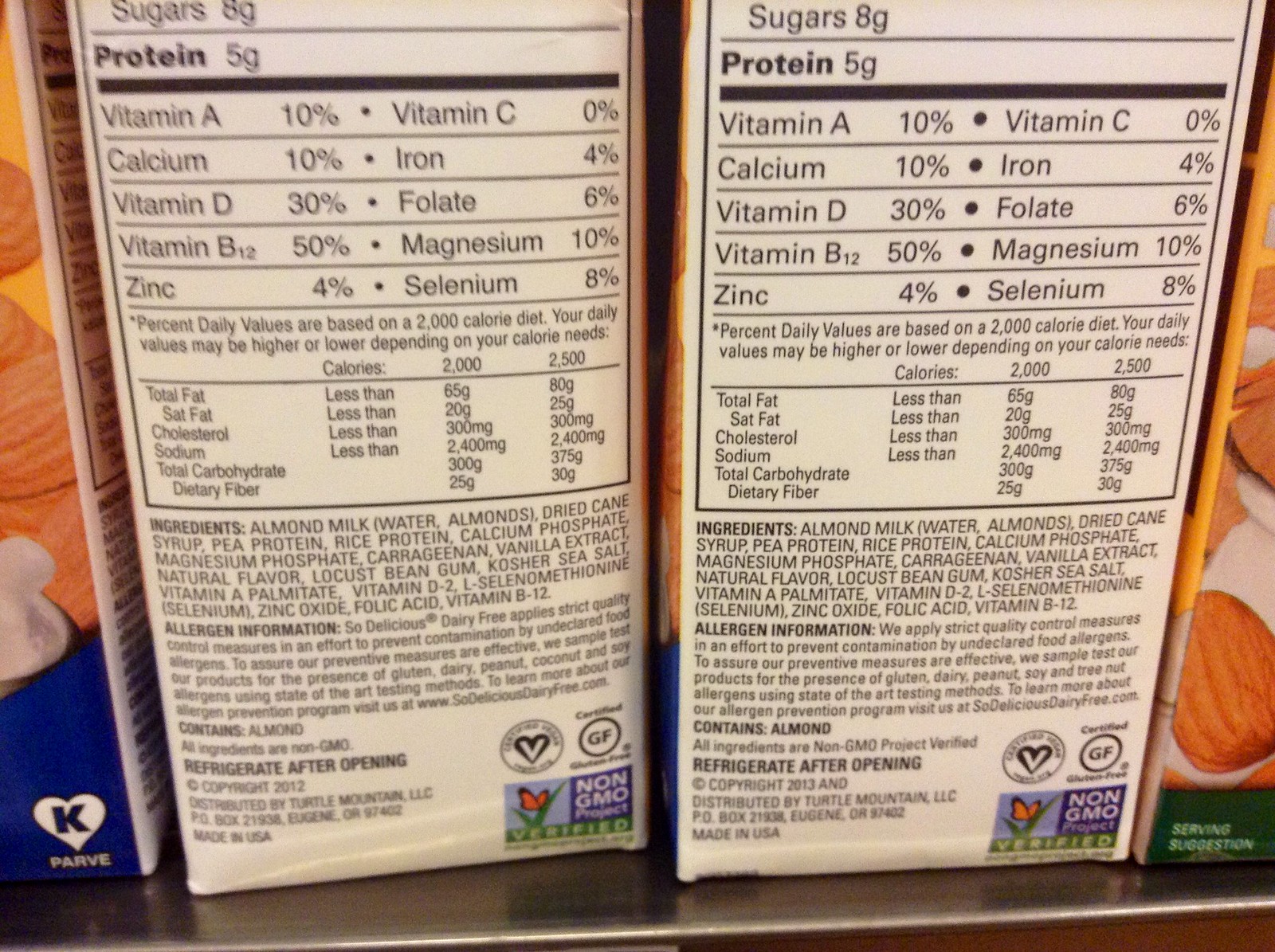This detailed color photograph captures multiple cartons of almond milk placed on a brown shelf. Two cartons are displayed with their front labels visible, while two are turned to reveal the nutritional facts on the back. The nutritional information lists 8 grams of sugar, 5 grams of protein, and various vitamins and minerals including vitamin A (10%), calcium (10%), vitamin D (30%), vitamin B12 (50%), zinc (4%), iron (4%), folate (6%), magnesium (10%), selenium (8%), and vitamin C (0%). The ingredients include water, almonds, dried cane syrup, with allergy information specifying the presence of almonds. Alongside the nutritional facts, the box mentions that it must be refrigerated after opening, and the product is non-GMO. The bottom features a small butterfly symbol representing the non-GMO project, and another icon indicating gluten-free certification. The overall visual has a reflective silver metal table beneath the cartons, providing a modern contrast to the brown shelf. This image, also showing a tan almond and a splash of white liquid representing milk on the carton, along with the Turtle Mountain, LLC distributor’s information, and a 2013 copyright, seamlessly captures the comprehensive details of the almond milk product.